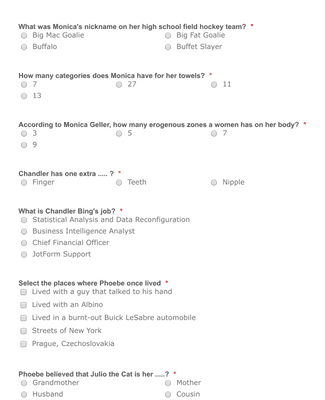This vertical image, captured from a computer or smartphone screen, showcases a multiple-choice quiz featuring questions about the TV show Friends. Each question is bolded in black, accompanied by a small red star-like circle to its left. Below each question are four possible answers, each preceded by a clickable circle dot. The answer choices are in a less bolded black font compared to the questions. 

The quiz includes the following:

1. "What was Monica's nickname on her high school field hockey team?" 
   - Options: Big Mac, Goalie, Buffalo, Big Fat Goalie, Buffet Slayer.

2. "How many categories does Monica have for her towels?" 
   - Options: 7, 13, 27, 11.

3. "According to Monica Geller, how many erogenous zones does a woman have on her body?" 
   - Options: 3, 9, 5, 7.

4. "Chandler has one extra finger, teeth, or nipple." 

5. "What is Chandler Bing's job?" 
   - Options: Fiscal analysis and data reconfiguration, business intelligence analyst, chief financial officer, job form support.

Additionally, there are two more questions with potential answers visible at the bottom, though they are not specified in detail. None of the questions have been answered, indicating the quiz is ready for interaction.